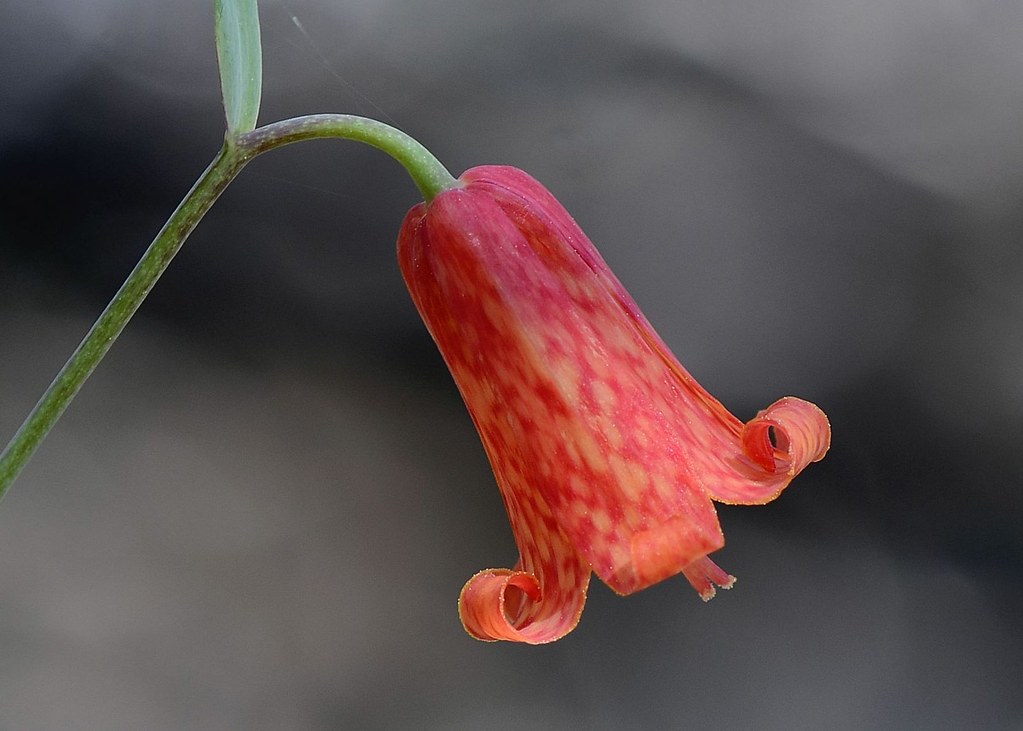The image features a photograph of a single flower stem against a slightly faded, textured gray background with deep dark gray segments. The flower's green stem extends from the left-hand side, curving towards the middle of the image. Connected to the stem is a single, thinner leaf, and a delicate thread, possibly a cobweb, links the leaf to the stem. The flower itself is bell-shaped and points downwards, with its vibrant reddish-orange petals curling back on themselves and exhibiting hints of yellow and pink. At the center of the flower, two small structures protrude, surrounded by yellow mottling, indicative of pollen. This detailed photograph captures the flower from a side view, emphasizing its natural elegance and invitingly pollen-rich environment.